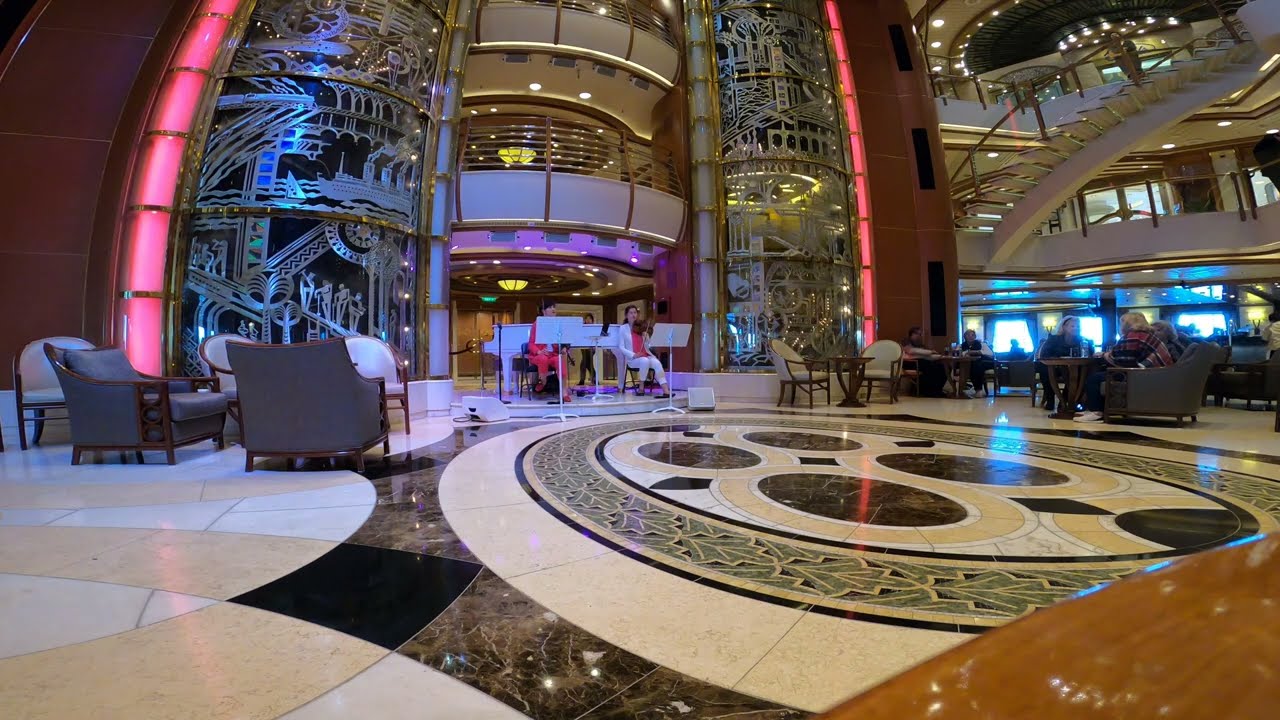The image depicts the opulent interior of a grand lobby, possibly of a hotel or cruise ship, characterized by its elaborate, shiny decor and tiled floor with intricate, ornate patterns. Dominating the scene is a large circular design on the floor, featuring concentric rings of light tan and dark brown hues, adorned with dark circles and diamonds. In the lower part of the image, the floor is dark brown with scattered white specks.

Central to the background, three musicians perform, one visibly holding a violin and dressed in white pants, a white jacket, and a pink top. Another musician sports a pink-red top and pants. They sit behind music stands, suggesting a live performance. Behind them are two-tiered floors with elaborate glass pillar windows, enhancing the luxurious ambiance.

On the left side, there are several lounge chairs, a mix of dark bluish-gray and white, all unoccupied. To the right, various people are seated around tables, seemingly engrossed in the concert. In the far-right background, bright lights illuminate what could be either display screens or gambling machines, contributing to the vibrant atmosphere.

Above and arching over the scene, there are several metal and silver decorative segments divided by brown strips. The top of the image is adorned with various floors, separated by curved edges and lit by multiple lights, adding to the space's grandeur. The upper-right corner reveals a staircase, hinting at more levels to explore. 

This lavish and possibly nighttime setting is enhanced by a large, illuminated arc at the top, filled with intricate silver and gold designs and what appear to be silhouette figures and letters, contributing to the overall majestic and bustling environment.